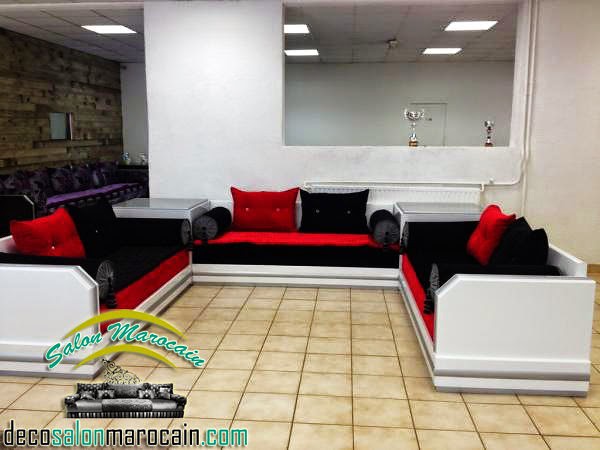This photograph captures an elegantly arranged sectional sofa displayed in a furniture showroom, branded under the distinctive Salon Marroquain logo and advertising the website DecoSalonMarroquain.com at the lower left corner. The dark-colored sofa icon, alongside its stylized script, hints at the luxurious nature of the furniture within. Dominating the scene, a U-shaped sectional sofa boasts white arms, backs, and rims, complemented by striking red and black cushions and pillows. This setup, resting on a beige pile floor, exudes modern comfort and style. The showroom features a brown tile design with fluorescent lighting, and an intriguing architectural detail—a wall opening showcasing a couple of trophies. A beige-brown wall flanks the background, enhancing the sophisticated ambiance with another black couch positioned strategically to complete the inviting look of this meticulously curated living room display.